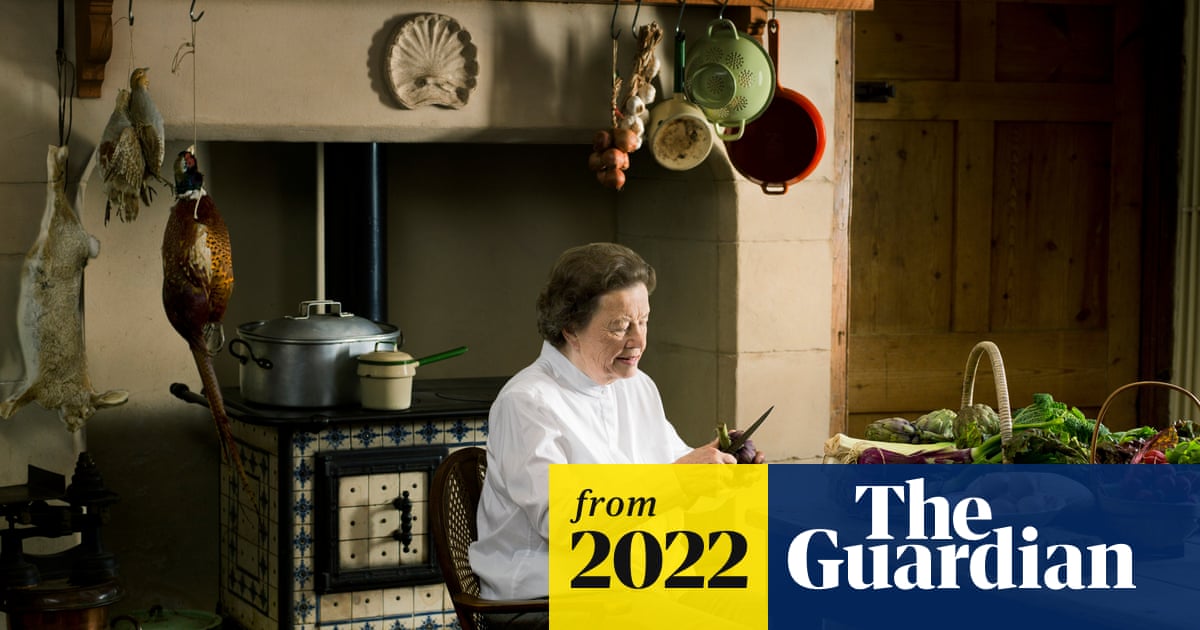The image captures a detailed scene of a vintage kitchen, prominently featuring an older woman, likely in her 60s or 70s, with short brown hair, who is wearing a white chef's shirt while sitting in a wicker chair and working intently with a paring knife to peel vegetables at a table. The table is scattered with produce, including artichokes and leafy greens stored in baskets. To the left side of the image, pheasants and a rabbit hang from hooks, adding a rustic charm. Behind the woman, an old-fashioned stove with blue and white tiles is visible, topped with a large silver pot and a smaller tan pot with a green handle. The background also shows a mantel adorned with various pots and pans hanging from the ceiling. The image is marked with a yellow rectangle stating "from 2022" and a blue rectangle with "The Guardian" in white text, indicating its source from The Guardian newspaper’s website.